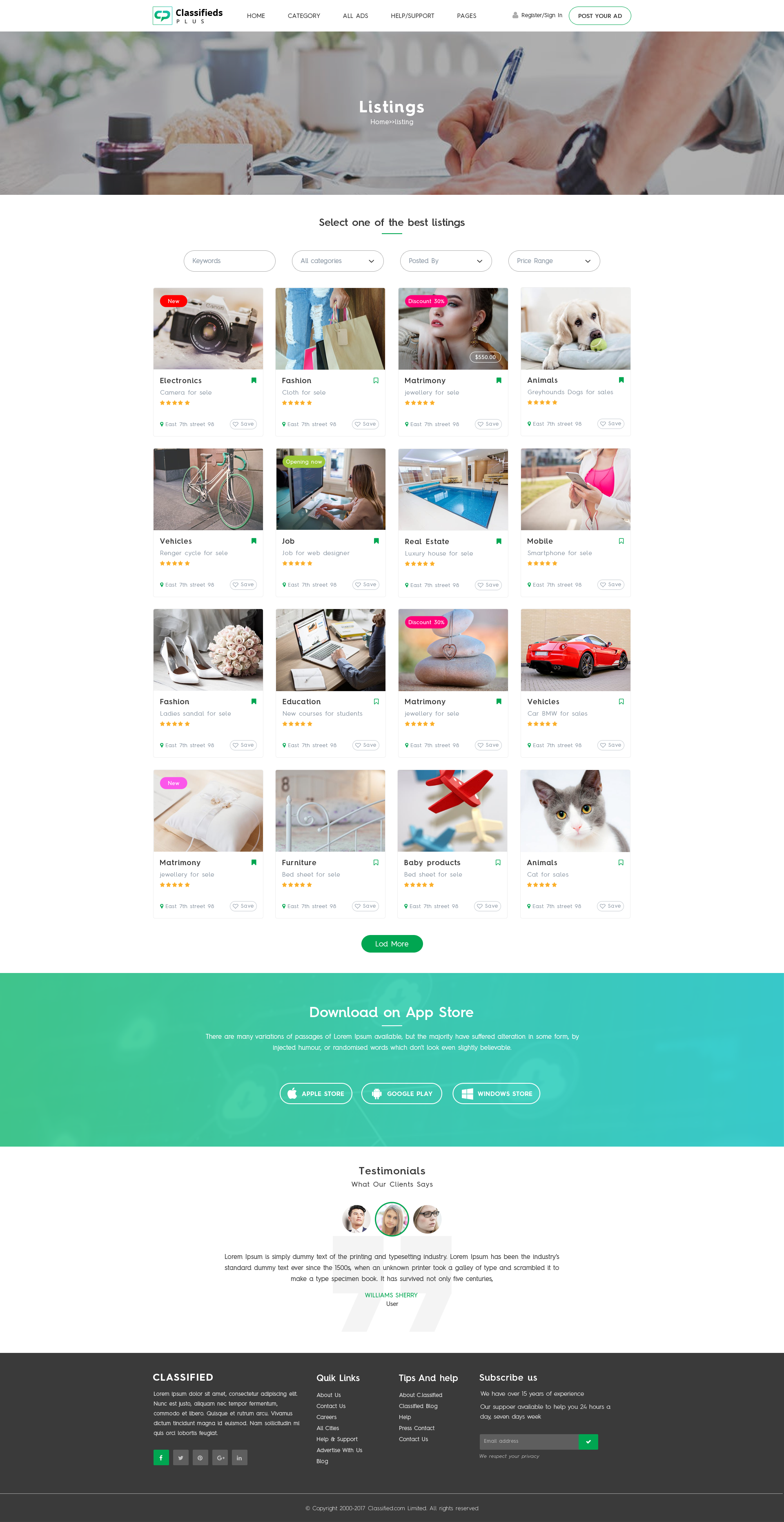The image depicts a detailed webpage layout for a classifieds website named "Classifieds Plus." At the top, the navigation menu includes options such as Home, Category, All Ads, Help/Support, Pages, along with buttons for Register/Sign In and Post Your Ad. 

The central section opens with a large header that reads "Listings" and below it, a subheader "Home" followed by "Listings" is displayed. Prominently featured beneath this is an image of a person writing with a pen on a desk, accompanied by the caption "Select one of the best listings."

Users can refine their search using the provided options for keywords, all categories, and filters for posting date and price range. Various categories are highlighted such as Electronics, Fashion, Vehicles, Jobs, Real Estate, Mobile, Education, Matrimony, and more. Each category is illustrated with an image; for instance, the Animals section showcases a picture of a cat labeled "Cats for Sale," while all listings show five-star ratings.

A green "Load More" button encourages users to browse additional listings. Furthermore, the bottom section of the webpage encourages users to download their app from the App Store and includes testimonials from current customers, adding a layer of user endorsement and credibility to the site.